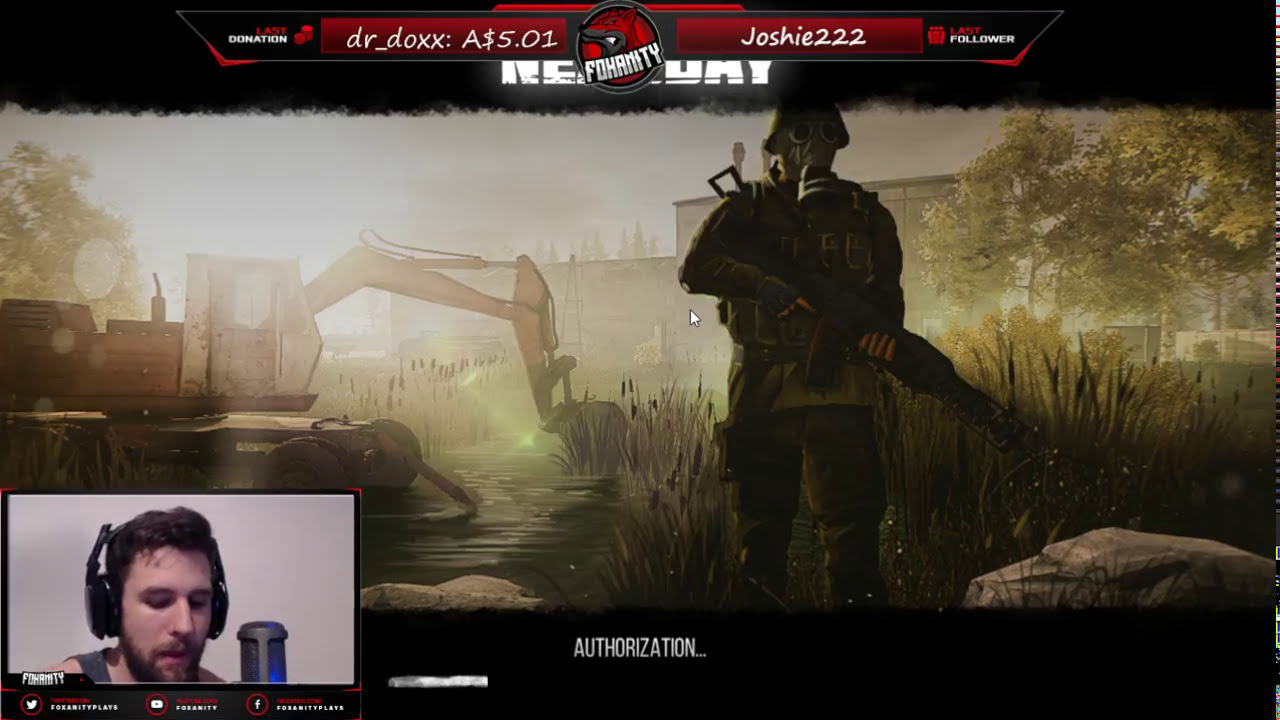In the image, we see a detailed scene of a gamer streaming a game, with his picture superimposed in the bottom left corner. The gamer, a young white male with dark brown hair and a beard and mustache, is wearing a large gaming headset and a gray tank top, though only one shoulder is visible. He is focused on the game, looking down towards a microphone in front of him, which features a noticeable blue light.

The main image showcases a surreal game environment. On the left side of the game screen, a large backhoe is situated in a watery, grass-laden area with cattails near its end, as if excavating a stream. To the right, a soldier-like game figure is standing, equipped with a gas mask and carrying a large gun. Surrounding the figure are boulders and trees, with what appears to be a building in the background. 

The entire image is framed with a black banner at the top and bottom. The top banner contains the text "authorization..." in white capital letters, indicating a loading or progress status. There is also a red inset banner displaying "doctor-docs doxxa $5.01 Joshie222." The detailed environment and focused gamer create an immersive representation of the gaming experience.